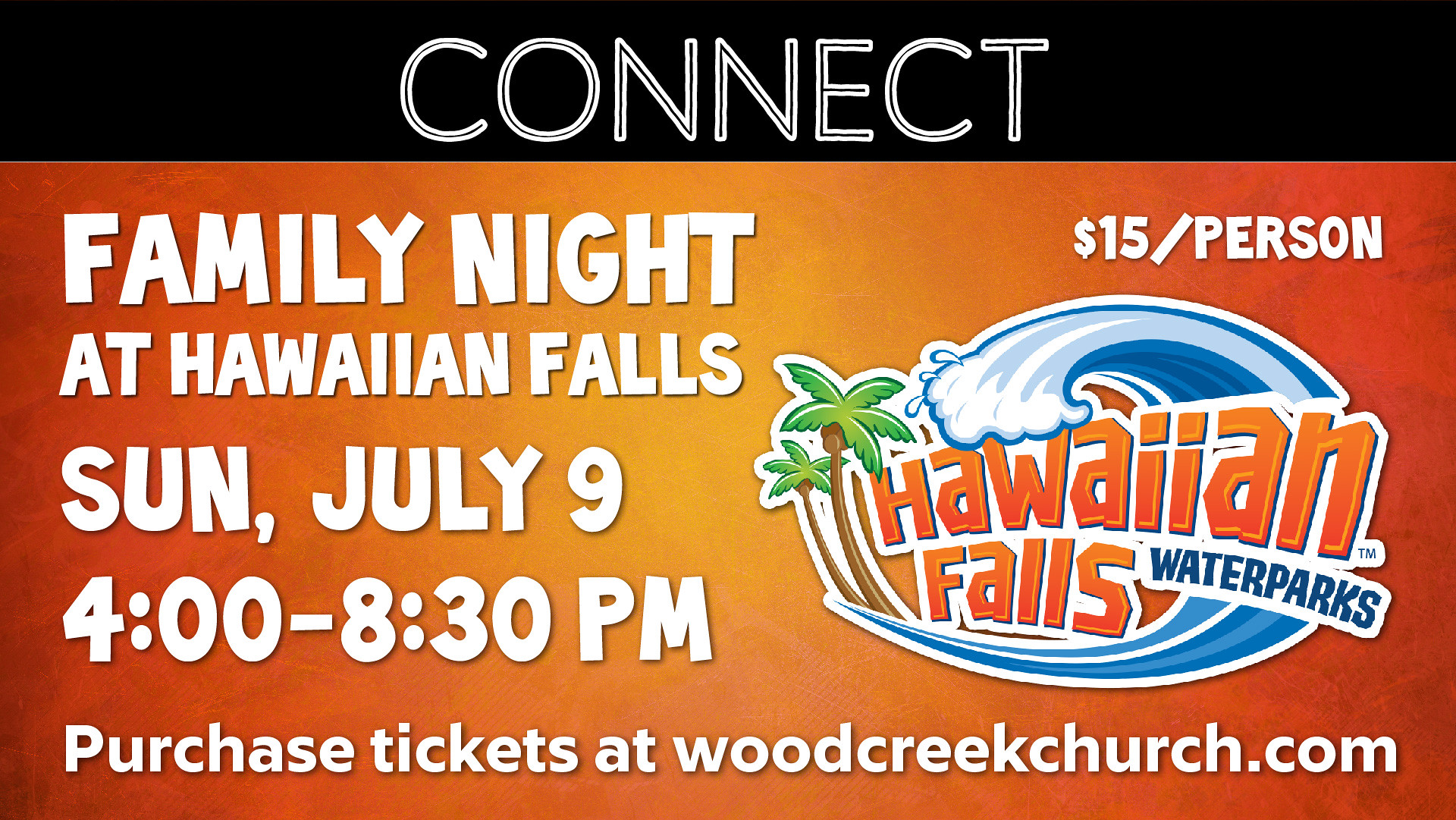This is a detailed advertisement for a family event. At the top, in white, capitalized letters against a black border, it says "CONNECT." Below, in white letters on a reddish-orange background, it announces "Family Night at Hawaiian Falls" on Sunday, July 9th, from 4:00 to 8:30 PM. Tickets can be purchased at Woodcreek Church for $15 per person. On the right side of the advertisement, there's a logo for Hawaiian Falls Waterparks, featuring blue and white waves and two palm trees with brown trunks and green fronds. The event details and logo are surrounded by a gradient background, transitioning from a lighter orange in the center to darker shades on the left, and the right side features a mix of orange, yellow, and red tones.